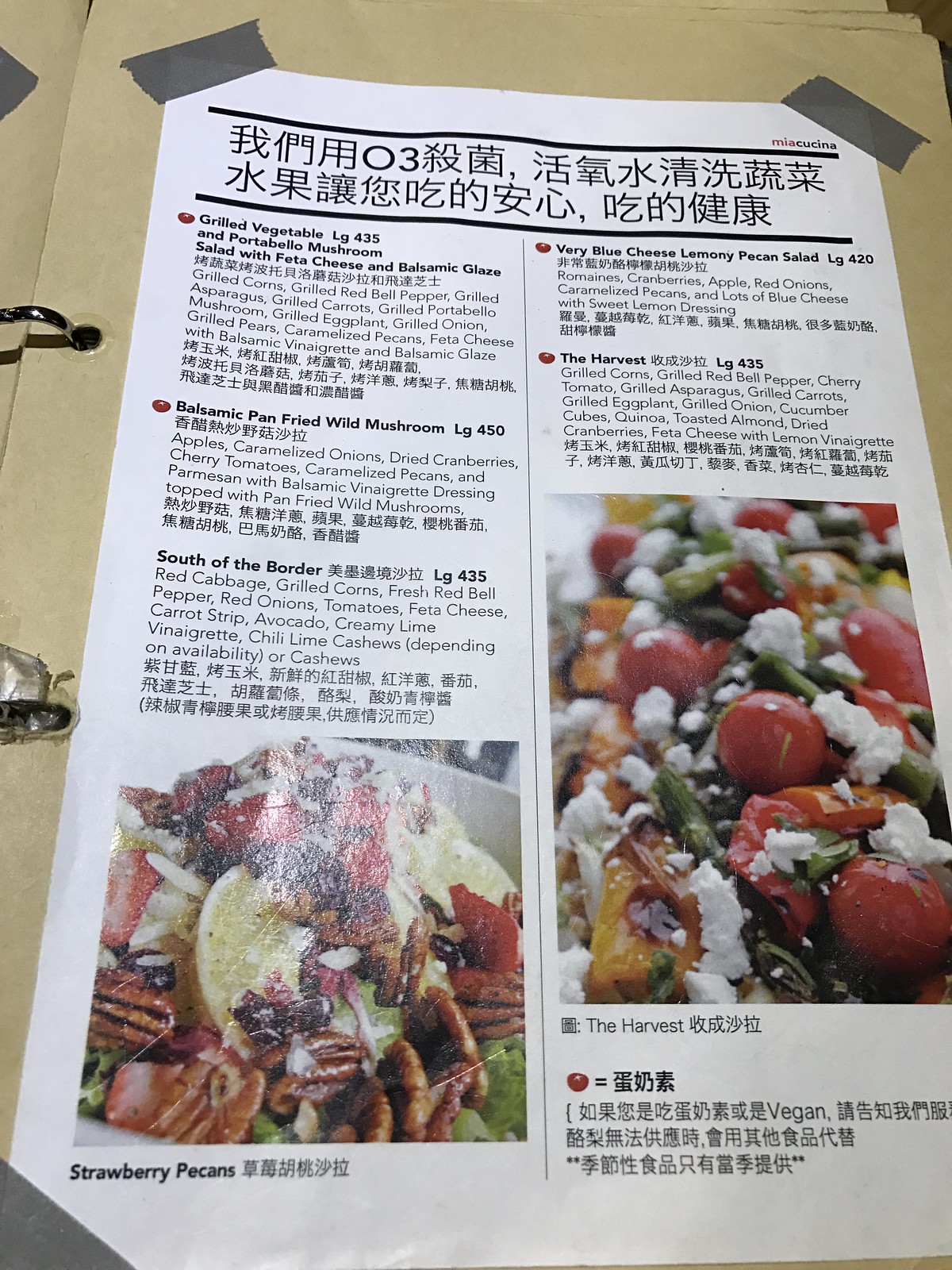The menu, presented on a clean white background with black text, displays dishes in both English and Chinese. It features two columns: the left column lists three menu items, while the right lists two. Each dish is named in Chinese and described in English, followed by a Chinese description. 

In the left column, the top dish is "Grilled Vegetables and Portobello Mushrooms with Feta Cheese and Balsamic Glaze", followed by "Portobello Mushroom Salad with Feta Cheese and Balsamic Glaze", each accompanied by detailed bilingual descriptions. At the bottom of this column, there's a photograph titled "Strawberry Pecans", showcasing vibrant strawberries and pecans.

The right column includes two menu offerings. The dish depicted at the bottom of this column is named "The Harvest", presenting a colorful array of cherry tomatoes, feta cheese, greens, and other salad ingredients.